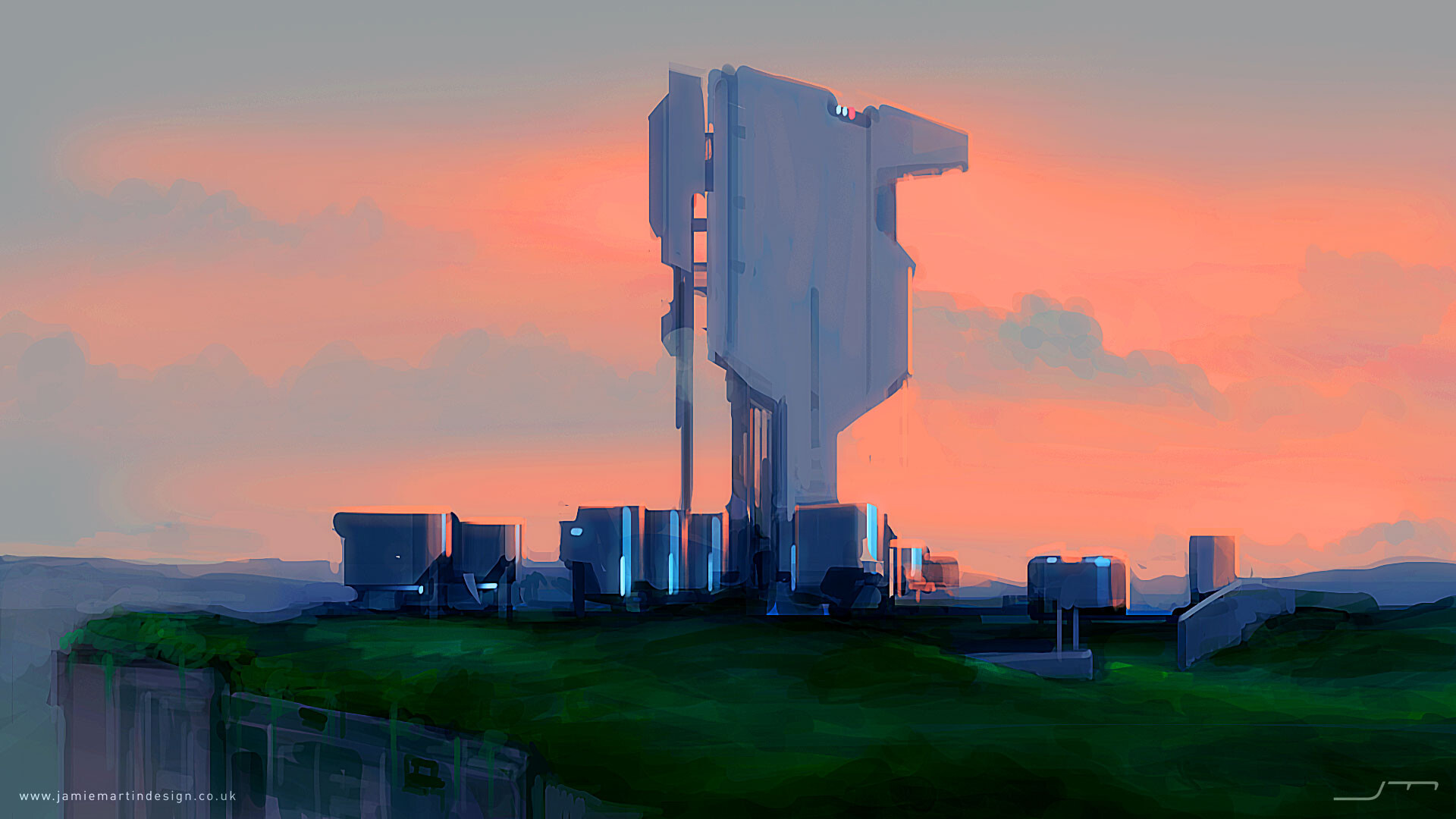In this detailed and striking image, we observe a highly futuristic scene that appears to be painted rather than photographed, presented with remarkable realism. Dominating the scene is a large, axe-shaped structure that towers above the rest, its upper reaches adorned with LED-like neon blue lights. This central structure is approximately five to six times taller than the surrounding high-rise, multi-story buildings, which themselves are distinctly modern and futuristic, featuring similar neon accents.

The landscape is intriguing, with a green grassy area that covers a man-made cliff face, composed of metallic panels that give a sense of an industrial complex. The cliff side features purple panels, possibly representing rock or other materials in this stylized illustration. The various smaller objects scattered around resemble slender, geometric-shaped electrical transformers, contributing to the sci-fi aesthetic.

The sky above is a mesmerizing gradient of pink and blue, adding to the otherworldly ambiance of the scene, reminiscent of environments from the Halo universe. This is further emphasized by the overall color palette and design elements, which evoke a sense of an alien yet familiar world. In the bottom left corner, the artist's signature "jamiemartindesign.co.uk" is visible, confirming the creation by Jamie Martin Design.